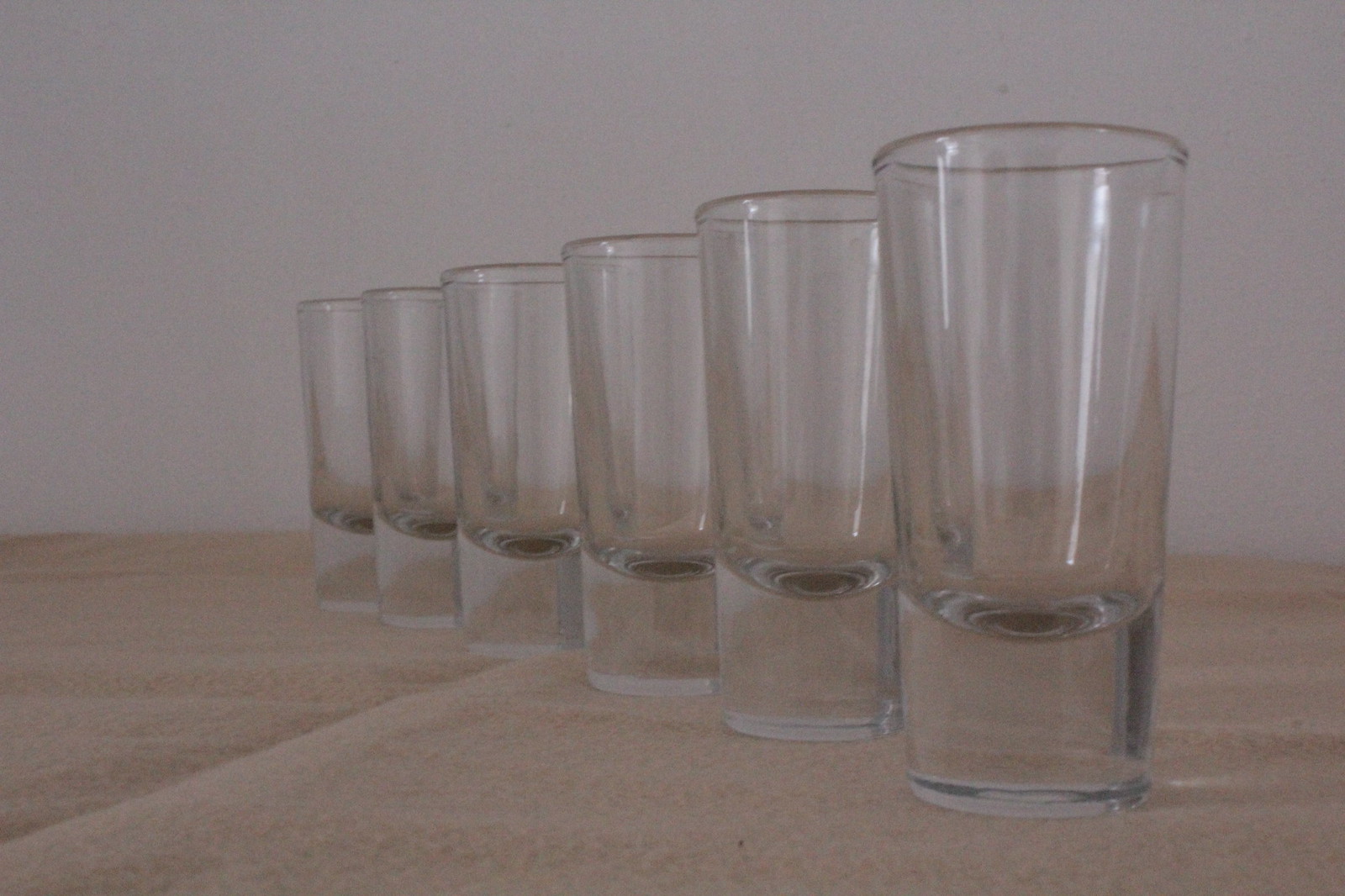This color photograph features six identical clear shot glasses, each with a thick bottom, lined up diagonally from the front right corner to the back left corner. The glasses gradually diminish in size due to the perspective, creating a dynamic visual effect. They sit on a beige-pink tablecloth that has some wrinkles, laid over a tabletop. In the background is a white surface that contributes to the overall dim lighting of the image. The reflection in the glasses hints at a sunny outdoor scene with shades drawn down, adding depth to the composition.